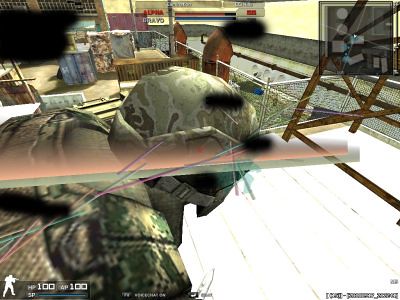The image is a low-definition screen capture from a video game, likely a war-themed game similar to Call of Duty. It depicts an indoor setting that could be a school, laboratory, airport, or military facility, characterized by the presence of tables with objects on them. In the foreground, the main focus is on a soldier crouching low to the ground, donned in futuristic combat armor with a light and dark green camouflage pattern. The soldier's helmeted head and upper torso are visible, suggesting they are sneaking around, possibly in search of a target. The background is somewhat blurry, with indeterminate shapes and a metal fence in the upper right corner. There is also a status display in the bottom left, indicating "100 hit points" and various game metrics. The periphery includes miscellaneous objects like a baby’s crib and a light pink tabletop. The detailed, but somewhat chaotic and blurred backdrop implies a high-intensity environment.